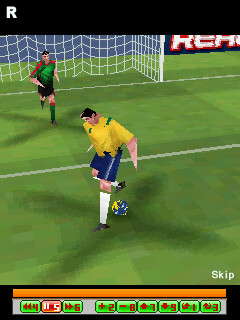This image captures a vibrant, classic soccer video game scene reminiscent of mid to early 90s PC games. Dominating the frame, a player in a yellow jersey with shoulder stripes and dark blue shorts, featuring a white stripe, prepares to kick a blue and yellow ball. His attire also includes white socks with green stripes and black shoes, with shin guards subtly visible, suggesting mid-action. Opposite him, the goalkeeper, dressed in a striking green and red striped shirt, black shorts, and dark green socks with stripes, rushes forward with one leg lifted, indicating dynamic movement. Both players are on a lush green AstroTurf field, with a white net behind the goalie. Insets display various game controls, such as play, pause, fast forward, and numeric toggles, along with a prominent orange progress bar at the bottom, possibly hinting at game playback or settings adjustments. At the top left, part of a scoreboard or interface is visible, partially showing "R-E-R" in white, red-outlined letters within a black rectangle. The screen's border includes black bars at the top and bottom, common in retro video game overlays.